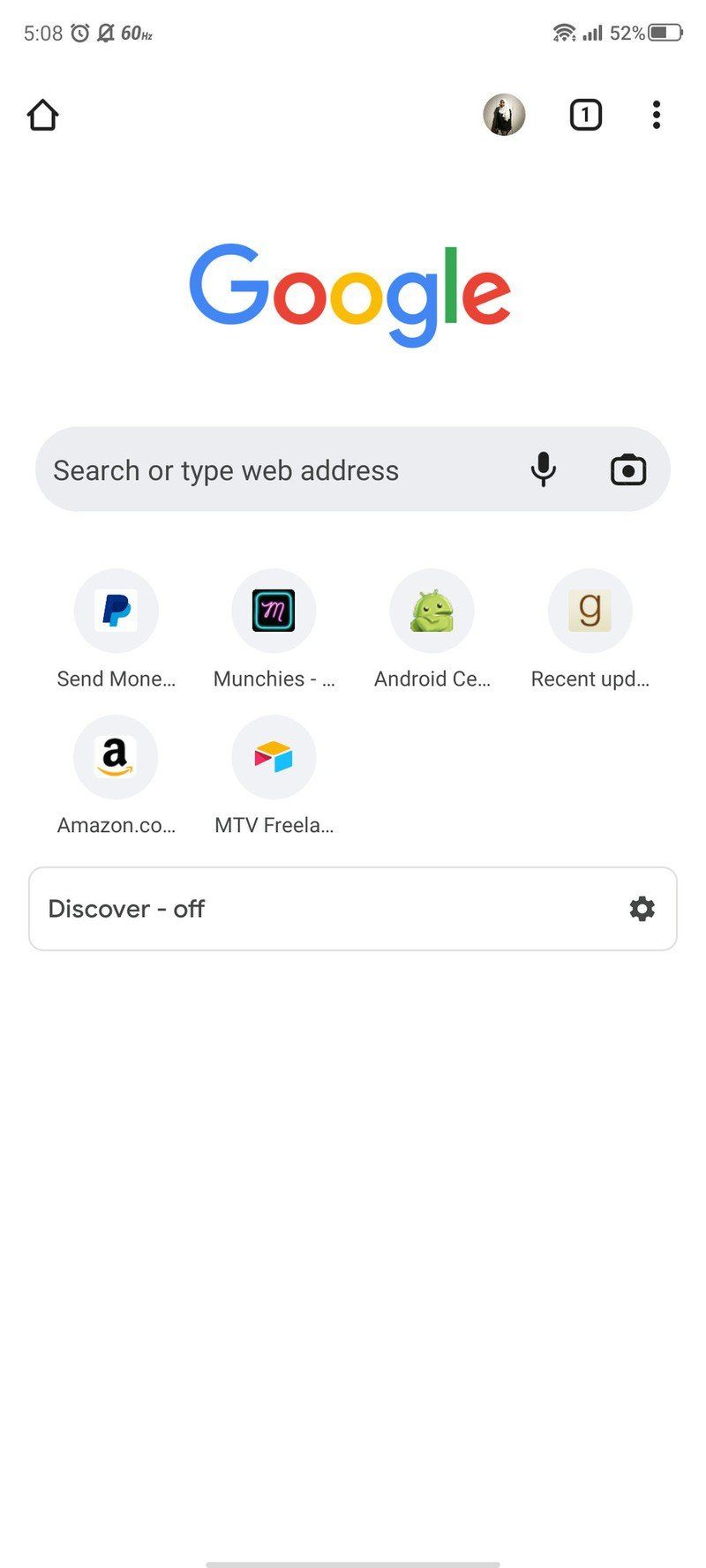This image is a screenshot of the Google application, possibly Google Chrome, displaying various interface elements in detail. At the top right corner, a half-full battery icon is shown, indicating a 52% charge with the left portion grayed out. Adjacent to the battery icon is the full strength indicator of the phone's signal. The top left corner shows the time as 5:08, accompanied by an alarm clock icon and a bell symbol with a line through it (likely indicating notifications are silenced). To the right of these, the screen refresh rate is displayed as "60 Hz."

Centered in the image is the Google logo, with each letter colored distinctly from left to right: the "G" in blue, followed by red, yellow, blue, green, red, and another red letter. Directly below the Google logo is a dark gray rectangular search bar that reads "Search or type web address." At the far right end of this bar are two icons in black: a microphone and a camera.

Below the search bar are six quick links displayed in two rows. The first row includes icons for PayPal, Munchies, and Android. The second row contains icons for G site, Amazon, and MTV.